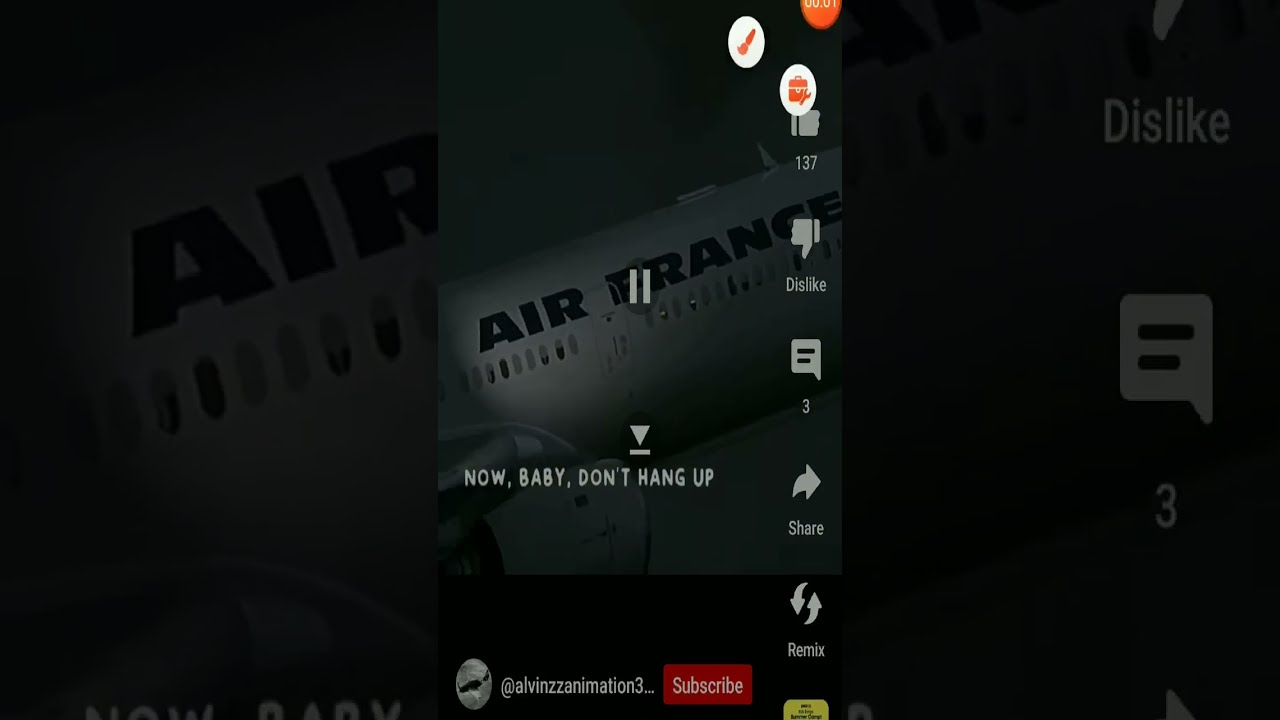This image appears to be a screen grab from a phone showing a paused video in a dark setting. Dominating the center is a vertical rectangle featuring a commercial airliner, likely an Air France jet, with a large pause symbol, indicating that the video is paused. Below the plane is a white text overlay reading, "now baby don't hang up," possibly hinting at a music video or song. 

On the right side of the screen, a vertical array of social media interaction icons is visible. These include a thumbs-up symbol with the count '137', a thumbs-down symbol labeled 'dislike', a chat icon with the number '3', an arrow labeled 'share', and a set of double arrows labeled 'remix'. Additionally, in the upper right corner, there are small white circles with orange icons, one featuring a paintbrush and another resembling a piece of luggage.

At the bottom of the image is a red button with the word 'subscribe' in white text, next to the account handle '@AlvinZZAnimation3'. The overall backdrop of the screenshot is dark, with the same image of the airplane blown up and mirrored in the background.